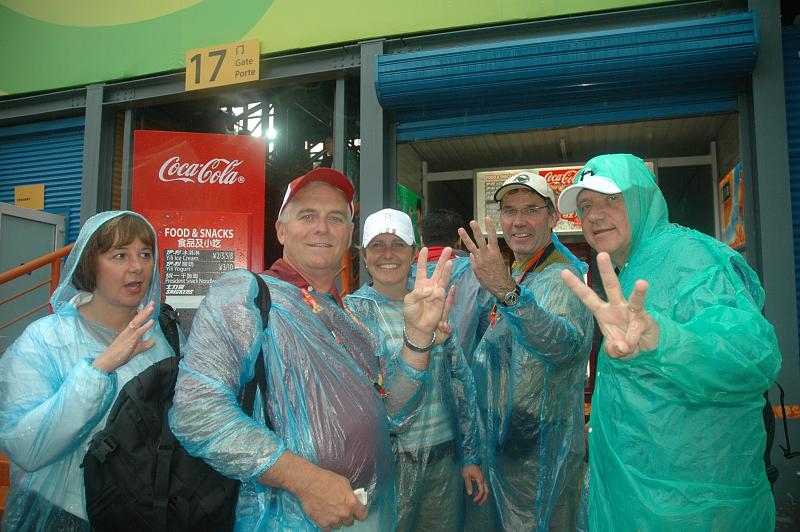In this vibrant group photo, five people are posing cheerfully outside a commercial building with a light green facade and a darker green swirl. The scene is lively, with additional details like blue drawn-up blinds and an orange handrail adding character. Each person is wearing a transparent, disposable greenish-blue rain poncho and a baseball cap, suggesting they might be co-workers on a break. Most of them, four out of five, are holding up their ring, middle, and index fingers, forming a "W" shape towards the camera. One gentleman, slightly diverging, is making the same gesture but with a backhand twist. A Coca-Cola sign in the background, advertising food and snacks, hints at a nearby shop, further indicated by the setting in what appears to be a bustling inner-city or downtown area. The woman on the left seems slightly distracted, seemingly unaware a photo is being taken.